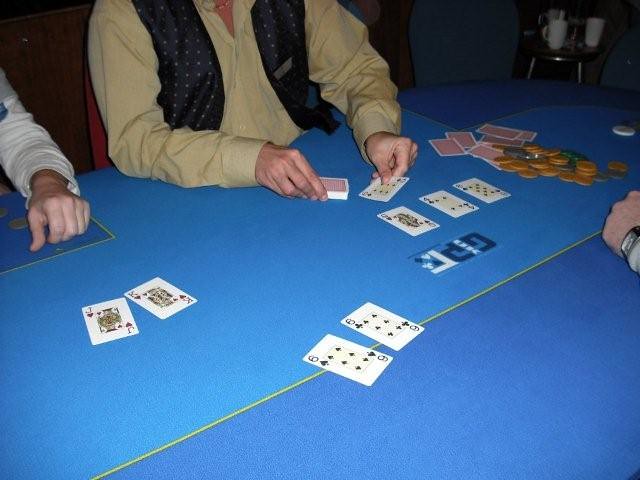In this detailed image, three individuals are engaged in a card game at a table featuring a blue surface accented by a distinct yellow line running down the middle. To the right of the table, two white cups are positioned. One of the players on the right sports a striking wristwatch, while the player on the left is partially visible, identifiable only by their white sleeve. The central figure, busy dealing the cards, is attired in a yellowish-brown shirt topped with a distinctive blue vest patterned with vertical dots.

The playing cards scattered across the table are predominantly red with white edges, and a collection of brown playing chips can be seen on the right side. Among the upturned cards, the Six of Diamonds appears twice in the center of the table. Nearby, the King of Hearts and the Jack of Hearts are also visible, while the rest of the cards remain obscured. The table itself bears a logo that is somewhat elusive, featuring two blue spots with a white section between them, intersected by a design of white and light blue streaks.